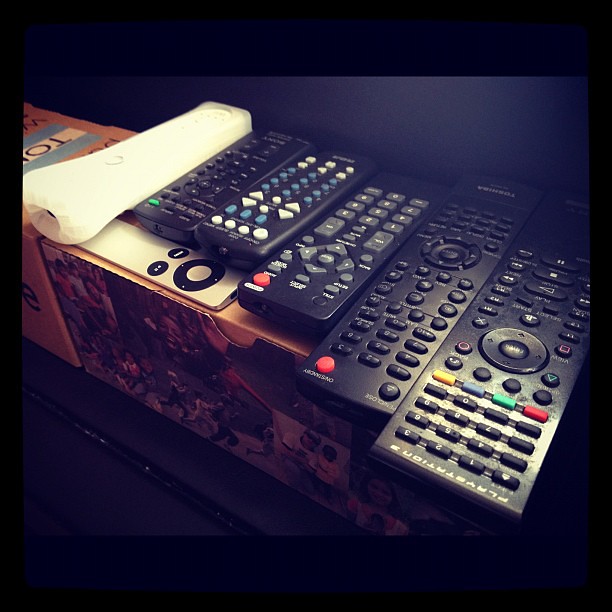This photograph, likely taken indoors at night based on the lighting, captures a diagonal arrangement of various remotes stretching from the top left to the bottom right corner of the image. The collection begins with a Wii remote on the far left, encased in a protective rubber cover. To its right, there is a black Sony remote distinguished by a singular green button amidst predominantly black buttons with white lettering. Next, another black remote features an array of white and blue buttons. Adjacent to it, a black remote showcases mainly gray buttons with white text and a standout red button. Continuing to the right, yet another black remote displays black buttons with white text, again with a prominent red button. The final remote on the far right, emblazoned with "PlayStation" at the top, features a mix of black buttons with white text and colored buttons—yellow, blue, green, and red—along with traditional PlayStation logo buttons. All the remotes rest on what appears to be a TV cabinet.